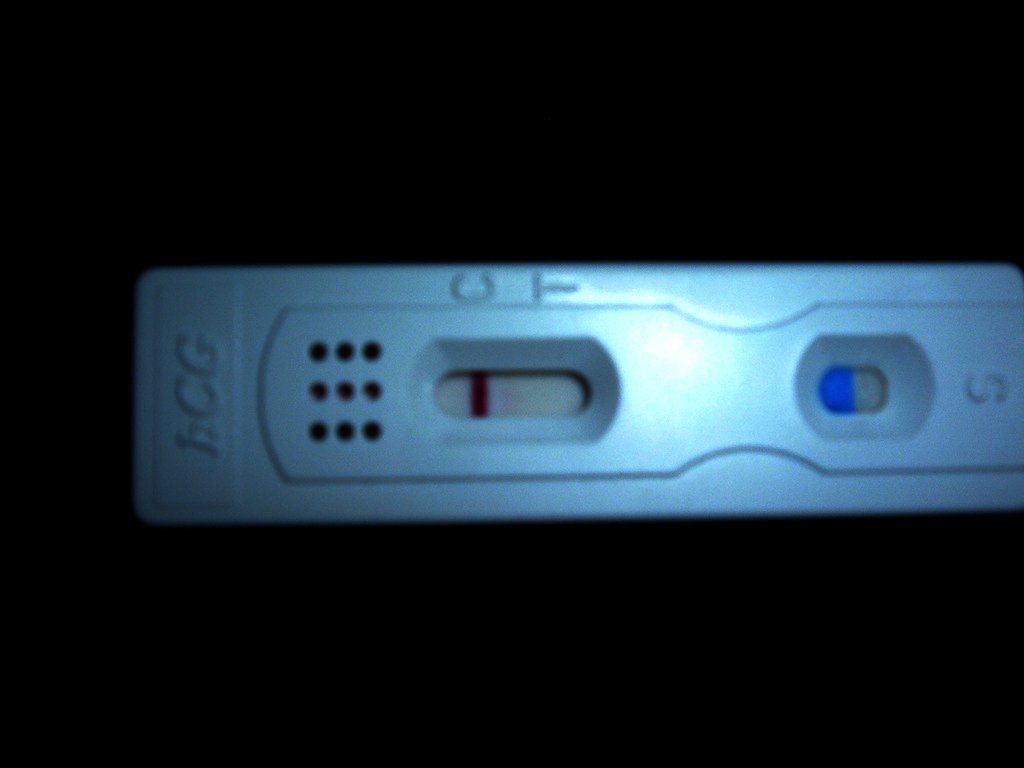This image displays a rectangular plastic device, likely a pregnancy test. The design features a classic meter with embossed letters indicating pregnancy status. The plastic casing prominently displays the acronym "HCG," possibly indicating the manufacturer. Near the meter, there are markings labeled "C" and "T." Below these markings, there's a button or indicator marked with an "S." The small display features a horizontal bar pointing toward the "C," though its exact meaning is unclear. At the top of the device, a speaker grill is present, suggesting it may provide audible feedback.